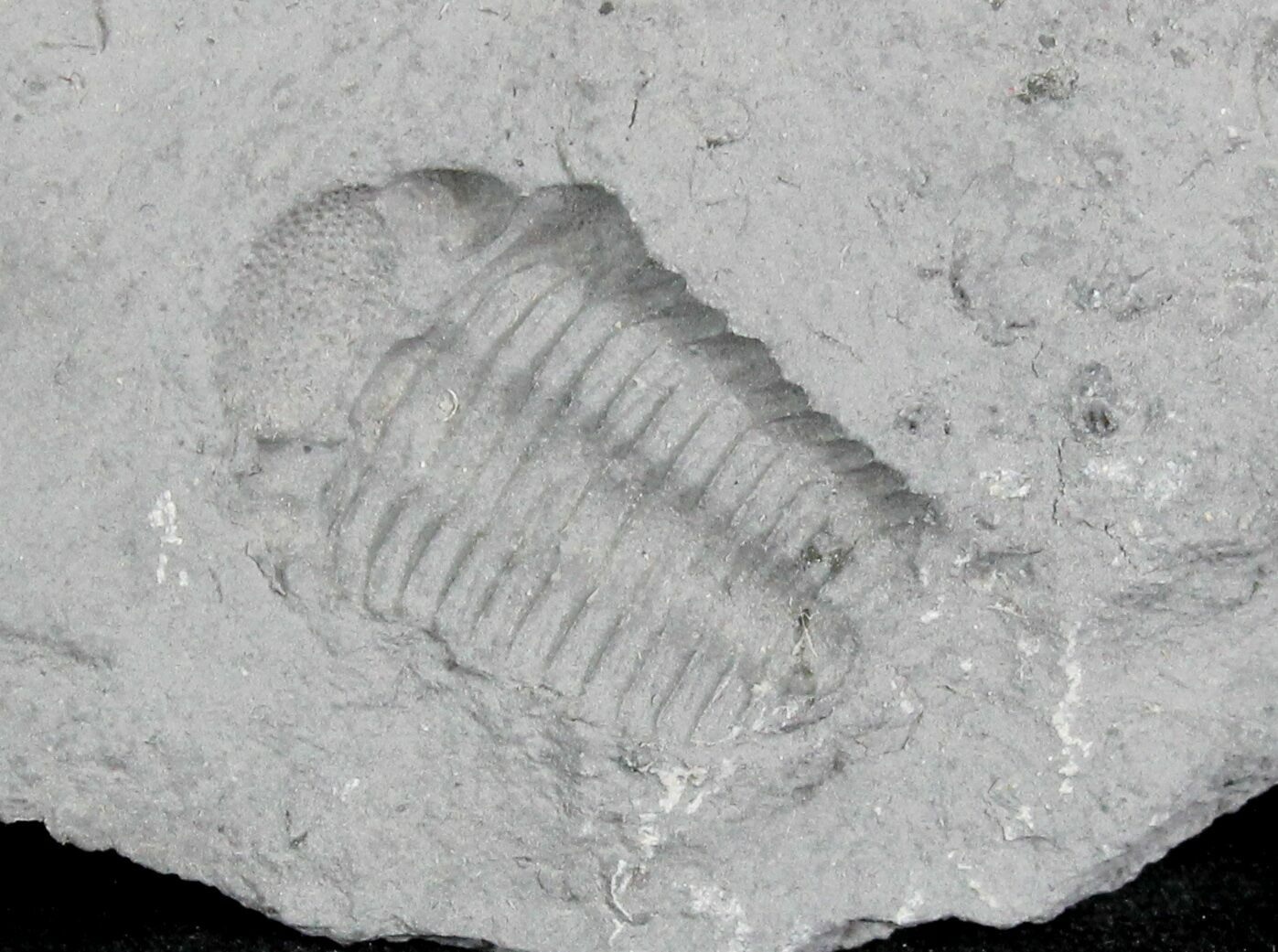This rectangular photograph, measuring approximately six inches wide and four inches high, showcases either a fossil or a plaster cast of a prehistoric aquatic creature embedded in a light gray stone with some gray specks and slight cracks. The creature is positioned diagonally towards the upper-left corner and features a rounded head adorned with small spikes and two pronounced eye-like bumps. Its body is composed of long, narrow rings, tightly compacted to form a scaly, segmented back. The fossil appears to be set against a dark, subtly sparkling background in the lower corners, accentuating the creature's detailed imprints, including horizontal lines and three distinct, elongated bumps with cavities in between.